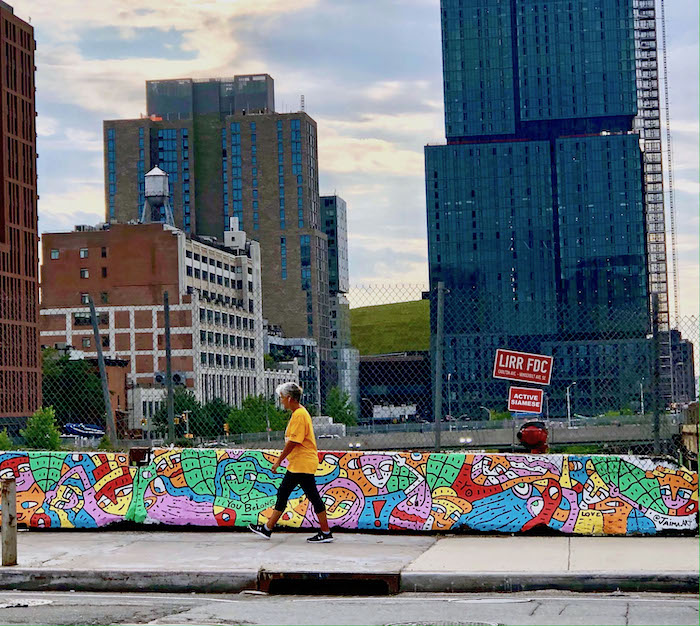In this outdoor photograph, we see a concrete sidewalk featuring large gray slabs where an older Caucasian woman with short gray hair walks. She is dressed in a yellow t-shirt, black leggings, and black shoes. Flanking the sidewalk is a concrete barrier wall topped with a gray chain-link fence. The wall is adorned with colorful and abstract graffiti and cartoon-like murals in shades of purple, green, blue, and red, some resembling human faces in a Picasso-esque style. Beyond the woman and the wall, the urban landscape showcases a range of tall, multi-story buildings. On the right stands a particularly tall high-rise with deep blue glass windows, still under construction, while to the left, a cluster of smaller buildings includes a red brick structure with white trim and a taller brown brick building. The sky above is a vivid blue with scattered clouds, adding to the vibrant urban setting.